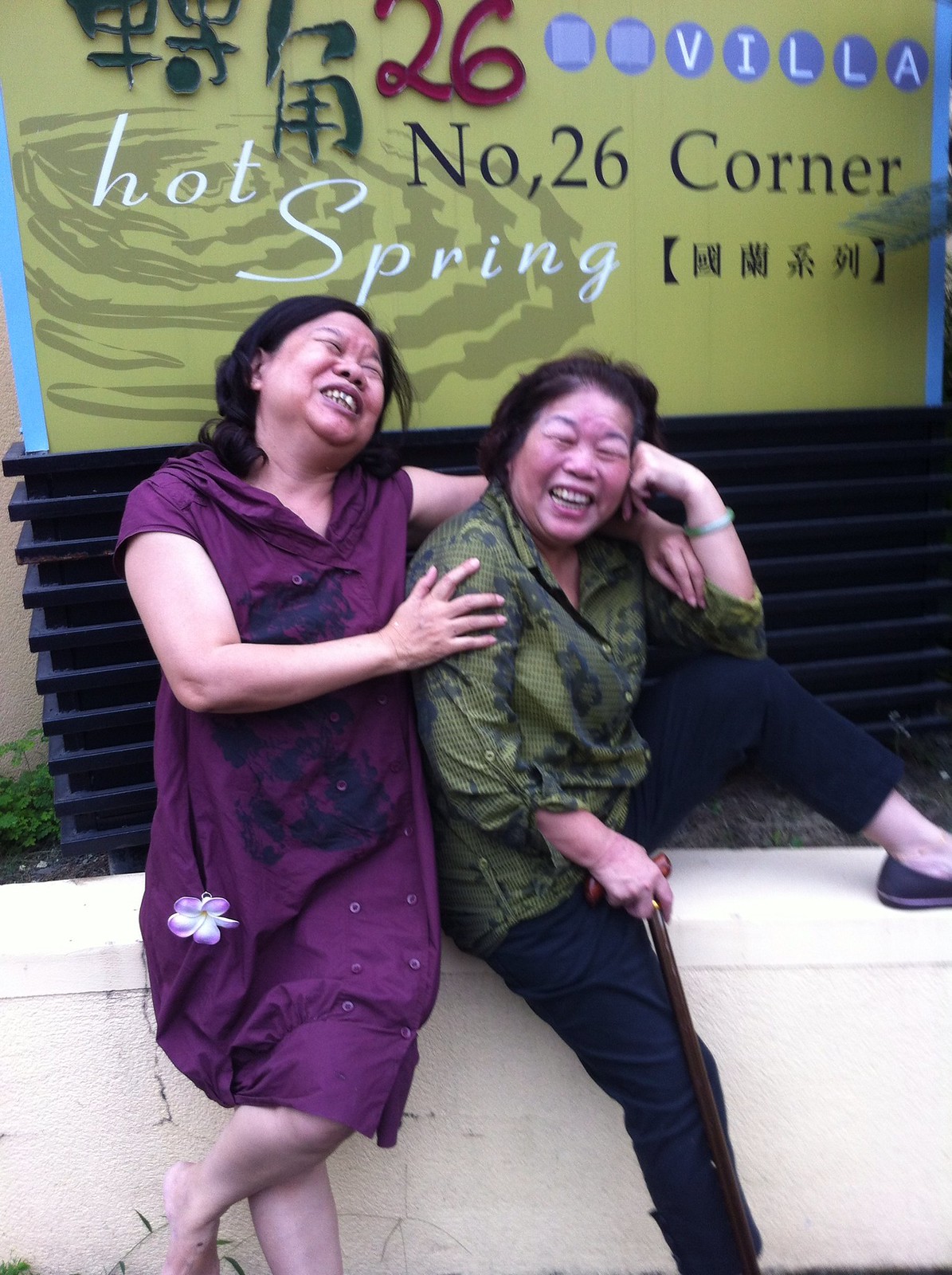In this vibrant image, two Asian women, possibly in their fifties or sixties, are captured in a moment of shared laughter, sitting on a white concrete barrier. The woman on the left, dressed in a purple floral dress that reaches just above her knees, throws her head back in laughter, with her right hand resting on the left bicep of the woman beside her and her left arm draped over the other's shoulder. The woman on the right sports a green button-down shirt and dark blue pants, seated with her left leg propped up on the wall and her right leg hanging over it. In her right hand, she holds a wooden cane, while her left hand supports her head as she leans on her knee, also laughing with her eyes closed. Both women have dark hair and their joy is palpable. Behind them, there is a yellow display board with the number 26 prominently displayed, along with the words "Villa," "Hot Spring," "number 26 corner," and some Asian characters, creating a colorful and lively backdrop. A small green plant adds to the serene ambiance of the scene.